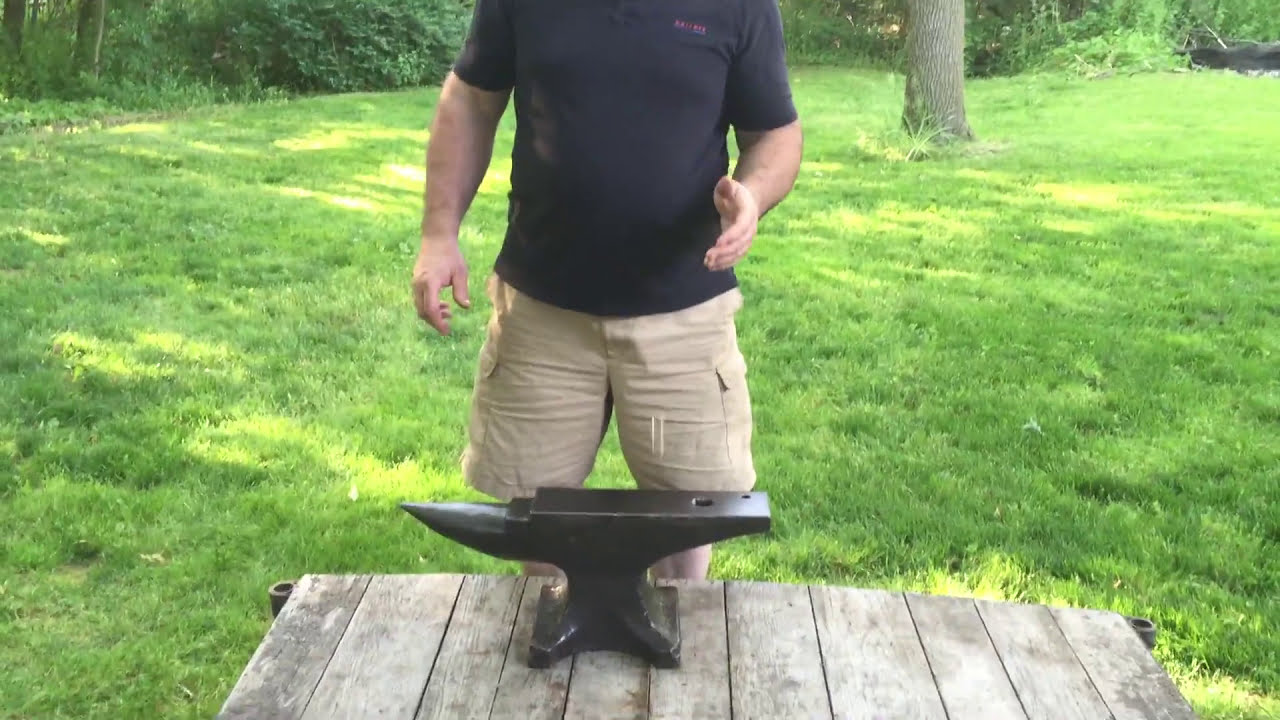The image captures a man standing outside in what appears to be a lush, green backyard or wooded area. His head is cropped out of the frame, leaving the view from his shoulders down to his knees. He is a white male, wearing a black t-shirt with a pocket and khaki-colored cargo shorts. The surroundings feature vibrant green grass, several trees, and bushes, with tree stumps and the bottom parts of trees visible. In front of him is a weathered wooden picnic table displaying a black, heavy metal anvil with a sharp edge on one end and a flat square top on the other. The background suggests a country setting, with elements like a walking trail and potential firewood hinting at a rustic lifestyle. Overall, the scene evokes a relaxed, country atmosphere, with the man seemingly poised to discuss or demonstrate the anvil on the table.